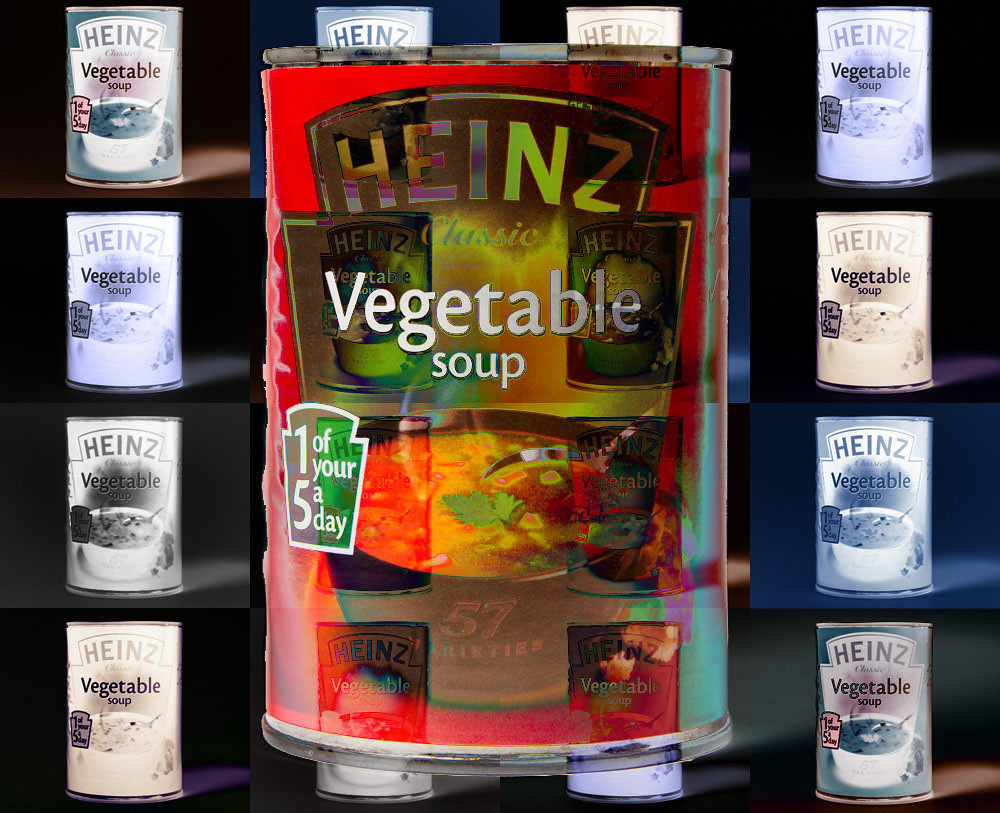The image is a detailed and artistic graphic design featuring a central can of Heinz vegetable soup, prominently displayed in its classic red color. The text on the can includes "Heinz" across the top, "vegetable soup" in white text, and a note at the bottom left stating "one of your five a day." The can is adorned with a silver steel cap and bottom. Surrounding this central can is a 4x4 grid of 16 smaller, square images of the same can, each tinted with different colors such as blue, green, purple, and yellow. These background images vary from grayscale to various color filters, creating a vibrant and dynamic collage.